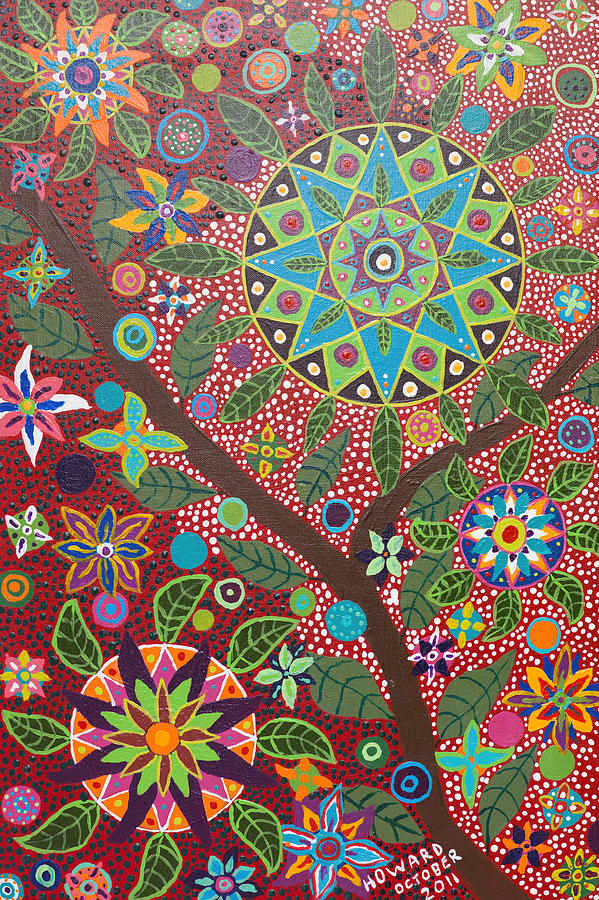This hand-drawn, portrait-oriented poster is a vibrant mosaic of psychedelic and geometric designs, reminiscent of a hippie aesthetic. Dominated by a colorful tapestry of leaves and flowers, the poster features a diagonal tree branch adorned with green leaves, detailed with simple vein lines. Surrounding this branch are multiple sacred geometry patterns, including multi-pointed stars and intricate mandalas, all brimming with clashing, bright colors like green, orange, pink, and blue.

The right half of the poster creates a dynamic contrast with its red background interspersed with white and black polka dots. Central to the composition, a large blue star-shaped flower is encased within a circle and surrounded by green leaves, notably enhancing the symmetrical design. Smaller circles, containing kaleidoscope-like patterns, are strewn throughout the piece, each framed by green leaves. The poster's intricate interplay of leaves, flowers, and geometric symbols results in a rich, symmetrically patterned visual experience.